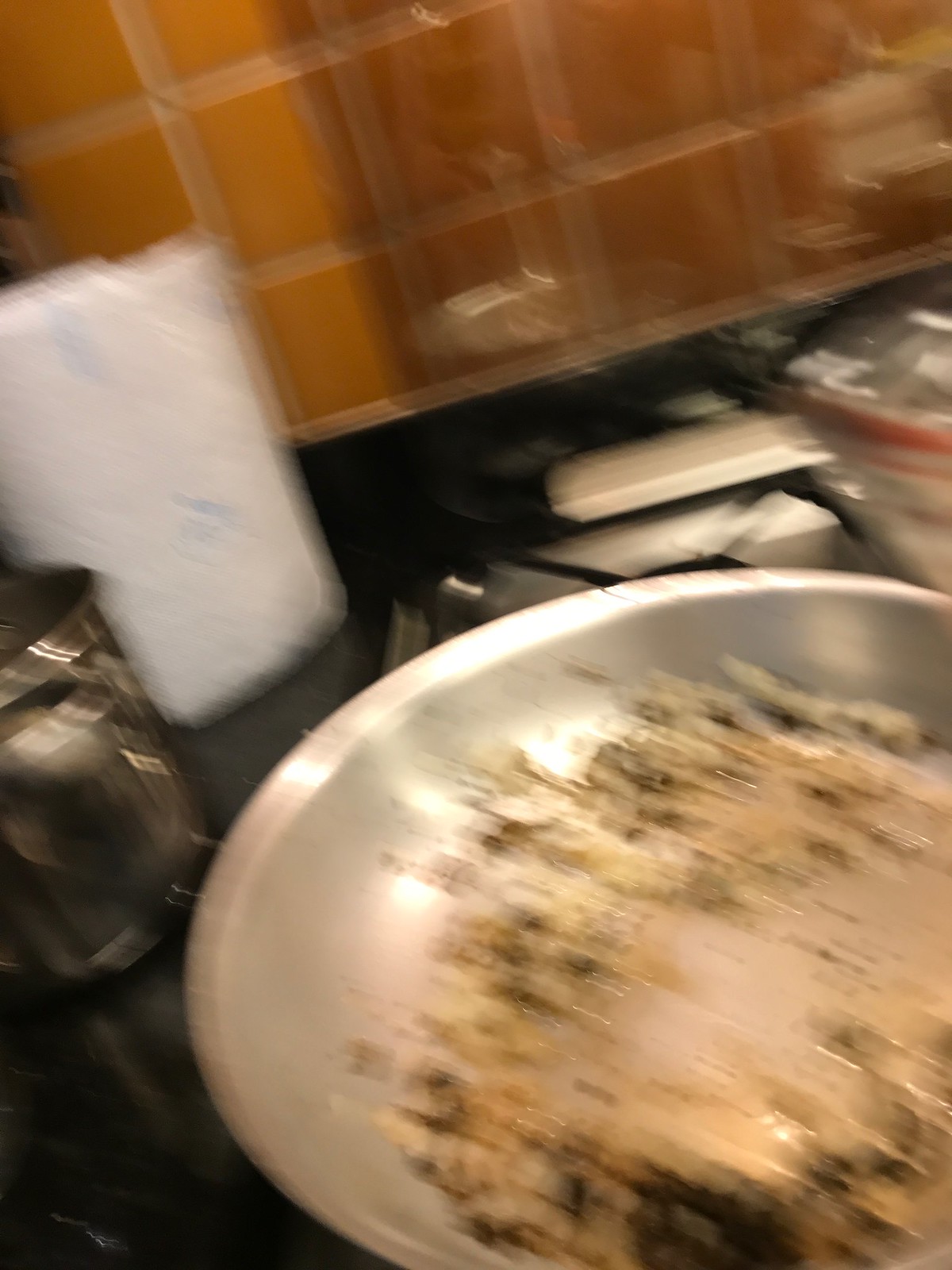This vertical, slightly blurred photograph captures a bustling kitchen scene during a cooking session. Dominating the lower right-hand quadrant of the image is a metallic pan filled with a brown substance, possibly ground beef or beans, actively cooking on a gas range. To the left of the stovetop, a roll of paper towels and a cylindrical container are easily identifiable, suggesting nearby kitchen essentials. Above the pan, a second metal grate burner is visible, consistent with typical gas stove designs. The backsplash provides a backdrop with its brownish-tan, salmon-colored square tiles. Another pot, though indistinct due to the motion blur, can be seen at the top right area of the frame, indicating a multi-tasking chef.